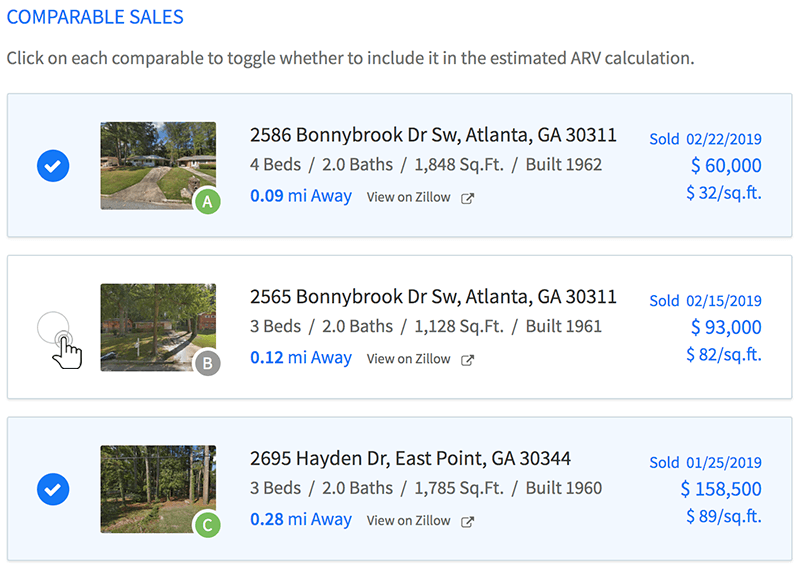**Image Description: Comparable Sales Listings on Zillow**

The image appears to be a screenshot of a webpage titled "Comparable Sales" from Zillow, which displays real estate listings used for property valuation. At the top, there is a note instructing users to "click on comparable to toggle whether to include it in the estimated ARV calculation." The term "ARV" (after repair value) is used in real estate to indicate the property's market value after renovations.

Below the header, there are three listings:

1. **2586 Bonnie Brook Drive SW, Atlanta, GA 30311**
   - **Status:** Checked (highlighted in blue)
   - **Thumbnail:** Street view of the house
   - **Details:**
     - Bedrooms: 4
     - Bathrooms: 2
     - Square Footage: 1,848 sq ft
     - Year Built: 1962
     - Price: $60,000 ($32 per sq ft)

2. **2565 Bonnie Brook Drive SW, Atlanta, GA 30311**
   - **Thumbnail:** None
   - **Details:**
     - Bedrooms: 3
     - Bathrooms: 2
     - Square Footage: 1,128 sq ft
     - Year Built: 1961
     - Price: $93,000 

3. **2695 Hayden Drive, East Point, GA 30344**
   - **Thumbnail:** None
   - **Details:**
     - Bedrooms: 3
     - Bathrooms: 2
     - Square Footage: 1,785 sq ft
     - Price: $158,500

The listings provide important details such as the number of bedrooms and bathrooms, size, year built, and the price per square foot. This information is used for estimating property values and comparing similar homes in the area.